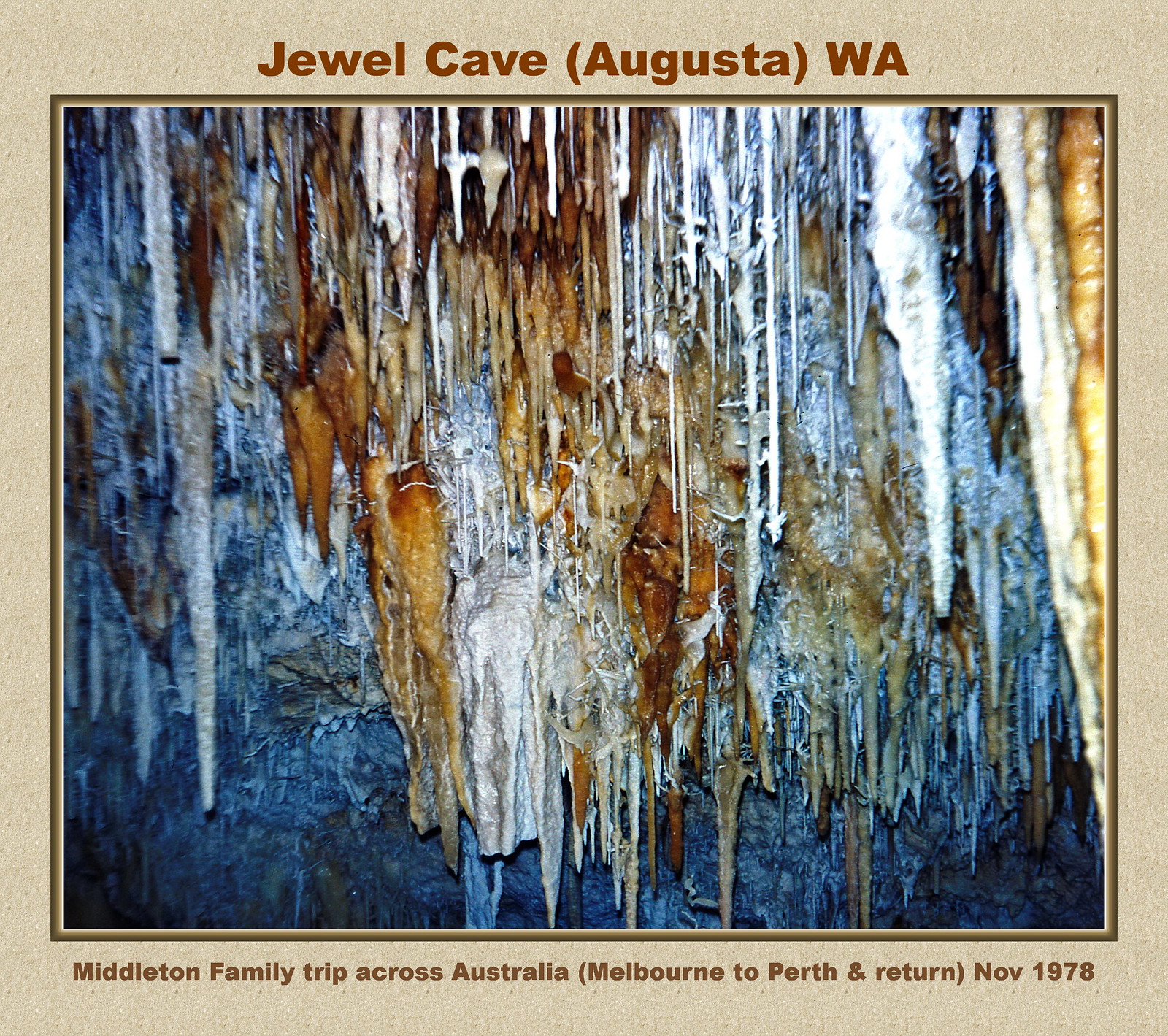This is a vintage landscape photograph, presumably a scanned image, featuring the interior of Jewel Cave in Augusta, Western Australia, taken during the Middleton family trip across Australia from Melbourne to Perth and back in November 1978. The photo depicts a series of stalactites of varying thicknesses and colors, primarily white, but also showing hues of rust, yellowy browns, and darker browns. These formations hang from the cave ceiling, resembling icicles against a bluish, rocky background that fades into darkness, suggesting the use of flash during the capture. The photograph is bordered with a light beige frame, with brown type captioning. The top reads "Jewel Cave, Augusta, WA," and the bottom declares, "Middleton family trip across Australia, Melbourne to Perth and return, November 1978," adding a nostalgic and personal touch to this compelling image of natural underground beauty.